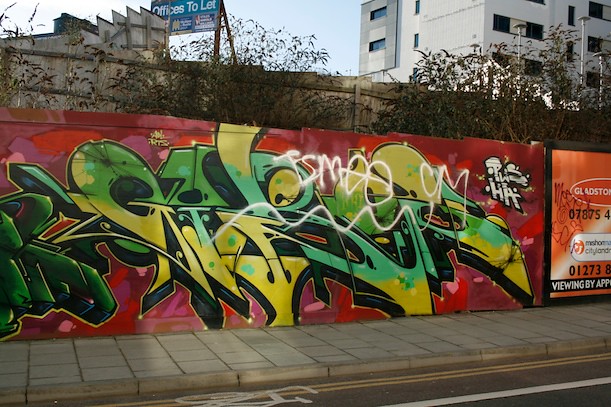The image is a daytime photograph of a street scene, framed horizontally. Dominating the scene is a large wall with intricate graffiti art, prominently featuring a red-toned background with blotches of dark and light reds. Bold, green and yellow text, shaded in black, sprawls across the wall, yet the lettering remains indiscernible. Additionally, white cursive spray paint over the top of the wall art forms unreadable squiggles and letters, including a discernible "T-S-M-E-E-C-M" with a squiggly underline, and "P-W-S" with "H-A" beneath it in the upper right corner. On the far right side of the wall, a yellow advertisement for Gladstone stands out.

In the foreground, a gray brick sidewalk is visible, transitioning into a bike lane that runs diagonally from the lower left to the upper right. Further back, above the wall, a wooden fence borders the scene with sparse trees in front. To the upper left portion of the picture, a billboard with a blue background reads "Offices Tillette" in white text. Finally, in the upper part of the image, a tall, white apartment building rises in the background, set against a clear blue sky.